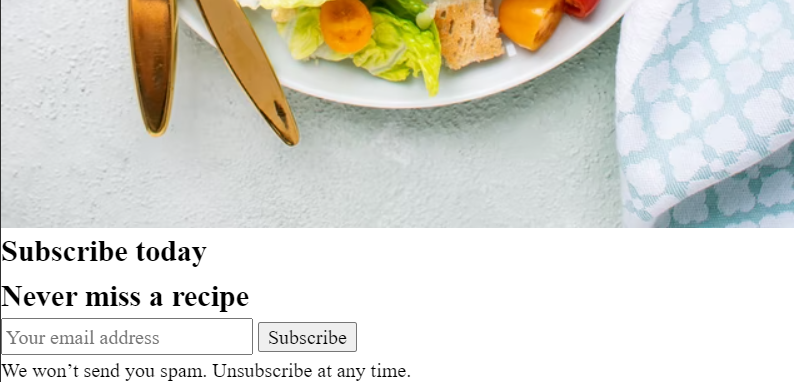The screenshot features a sign-up overlay soliciting email subscriptions for updates and recipes. The top portion displays a visually appealing banner, adorned with a pale blue tablecloth, a blue and white napkin, and the lower edge of a plate laden with a fresh salad. The salad comprises lettuce, croutons, and cherry tomatoes, accented by a couple of gold-handled utensils positioned to the left. Beneath this image, bold black text instructs users to "Subscribe Today," followed by "Never miss a recipe," which is then succeeded by an input field prompting users to enter their email address. A prominent "Subscribe" button invites action, accompanied by a reassurance that they "won't send you spam" and that users can "unsubscribe at any time." This call to action emphasizes the convenience and benefits of joining the mailing list while offering visual enticement with the tantalizing image of a salad.